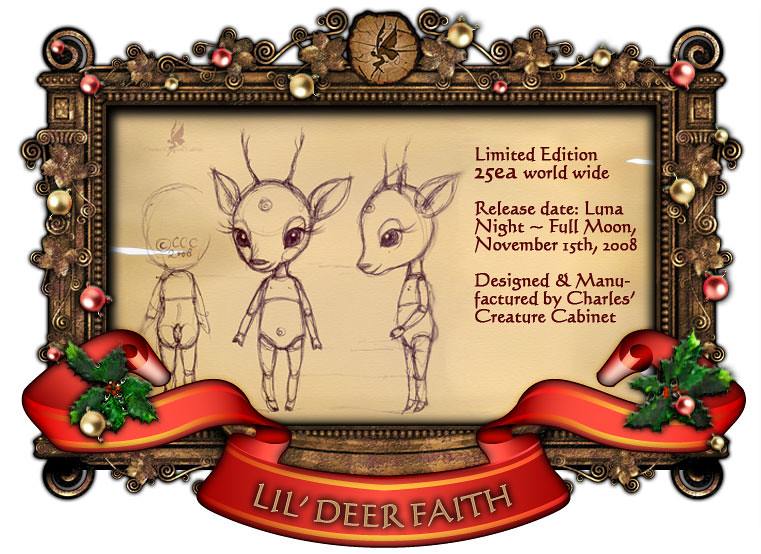This image showcases an ornately designed frame that radiates opulence with its gold and bronze hues. The frame is adorned with intricate swirls and curls, interspersed with red and gold bulbs that add a touch of vibrancy. Enhancing its lower section, a red banner embellished with gold stripes on the top and bottom edges prominently displays the inscription "Lil Dear Faith."

Enclosed within this elaborate border, the image boasts a beige background. Positioned on the right-hand side, informational text denotes this piece as a "Limited Edition, 25 each worldwide," with a release date of "Luna Night, Full Moon, November 15th, 2008," and crediting it as "Designed and manufactured by Charles's Creature Cabinet."

Dominating the left portion of the frame, the artwork features three extraterrestrial-like yet humanoid creatures. These beings, characterized by their large, expressive eyes, pointy ears, and delicate antennae, assume varied poses: one facing backward, another in profile, and the last gazing directly at the viewer. This captivating trio lends an air of mystique and otherworldliness to the entire composition.